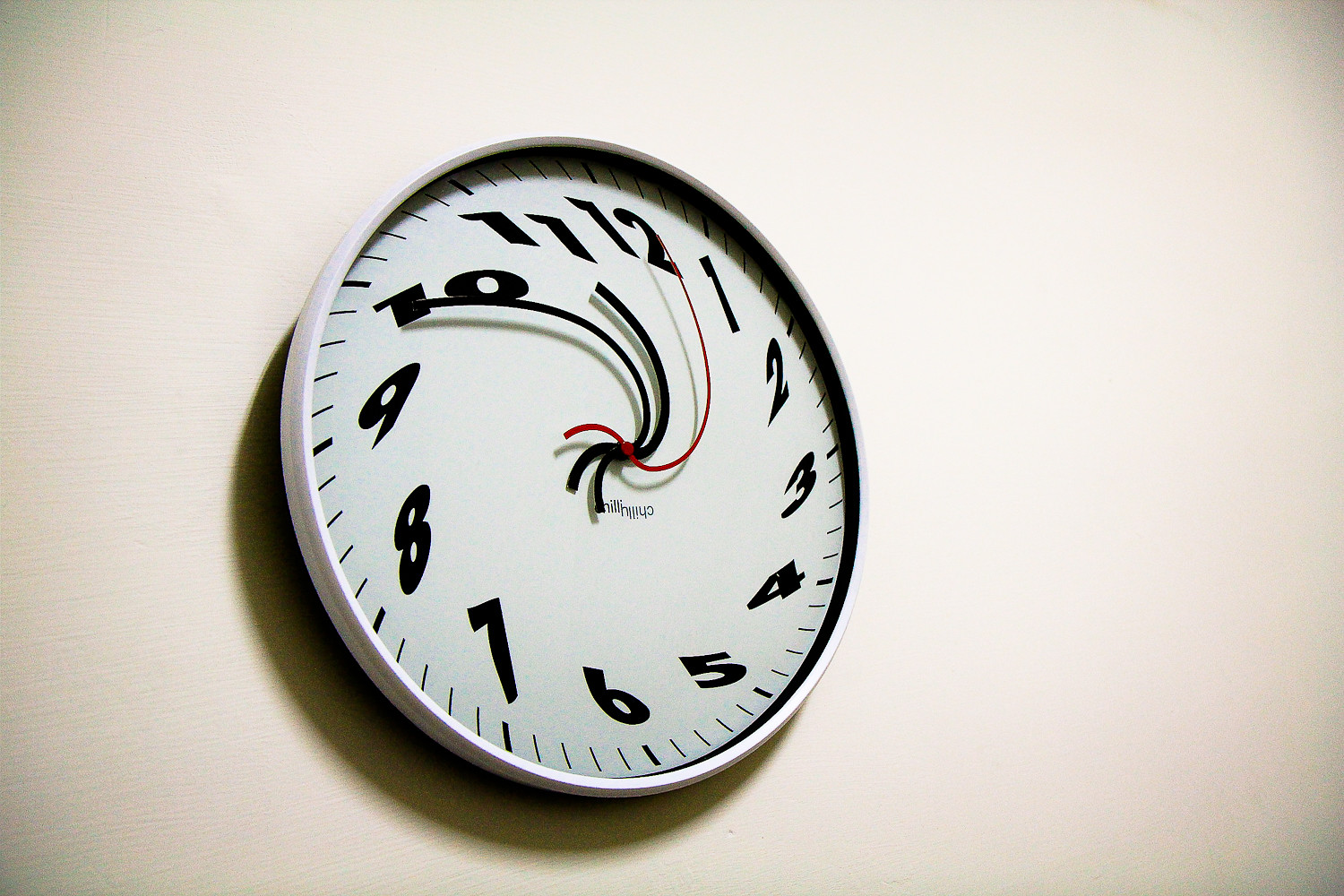A photograph captures a distorted white clock mounted on a pristine white wall. The clock's face is whimsically twisted, reminiscent of a funhouse mirror, with black, swirling numbers that defy conventional symmetry. The clock features two thick black hands and one slender red hand, which collectively obscure some gray-textured font beneath them. The circular frame of the clock, also white, casts a subtle but discernible shadow on the wall behind, emphasizing the clock's three-dimensionality. The corners of the image display a faint gray shading, adding depth to the otherwise minimalist composition, which centers solely on the quirky, eye-catching timepiece.